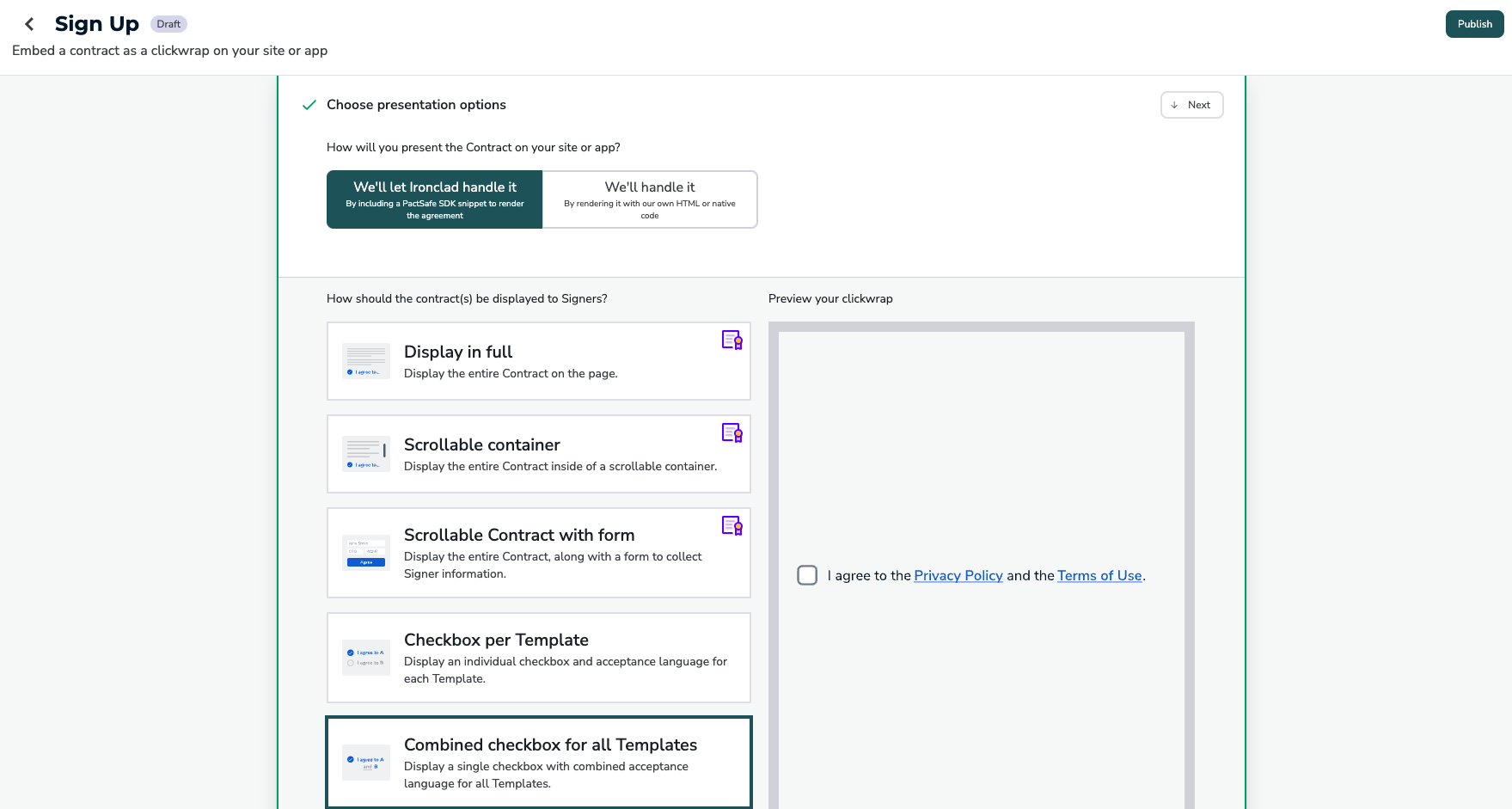This image depicts a sign-up website focused on guiding users on how to embed a contract as a clickwrap on their site or app. The background is predominantly gray. At the top left corner stands the bold black text "Sign Up" accompanied by a back arrow on its left and the word "Draft" on its right. Directly below, a brief instructional text reads, "Embed a contract as a clickwrap on your site or app."

On the main section, the heading "Choose Presentation Options" is highlighted with a green check mark. Below this, a question is posed: "How will you present the contract on your site or app?" Two options are presented for the user to choose from: "We'll let Ironclad handle it" and "We'll handle it." The selected option, indicated in green, is "We'll let Ironclad handle it."

Further down, various presentation modes are listed:
1. Display in Full
2. Scrollable Container
3. Scrollable Contract with Form
4. Checkbox per Template
5. Combined Checkbox for All Templates (this option is currently highlighted).

To the right, there is an area with a checkbox stating, "I agree to the Privacy Policy and the Terms of Use," allowing users to consent to these terms by marking the checkbox.